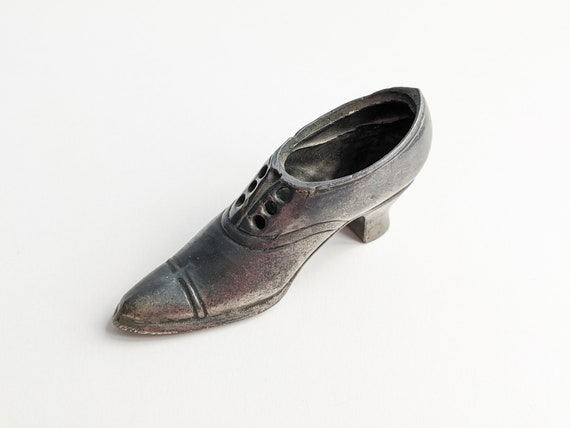The image depicts a unique shoe that appears more like a sculpture due to its heavy, metallic appearance and distinct characteristics. The shoe, facing left against a completely white background, features a very pointed toe and a low heel, giving it an antiquated look reminiscent of footwear from a century ago. Its overall color is dark brown, though it is worn down near the sole, revealing a lighter brown from extensive use. The shoe has six perfectly round holes for laces, accentuating its metallic facade, with no eyelets, further contributing to its sculptural, garden-like quality. Intricate lines adorn the top and bottom portion of the shoe, adding to its complex and artistic design. The interior appears to be made of leather yet maintains a metallic semblance, blending rustic and industrial elements into one intriguing piece.